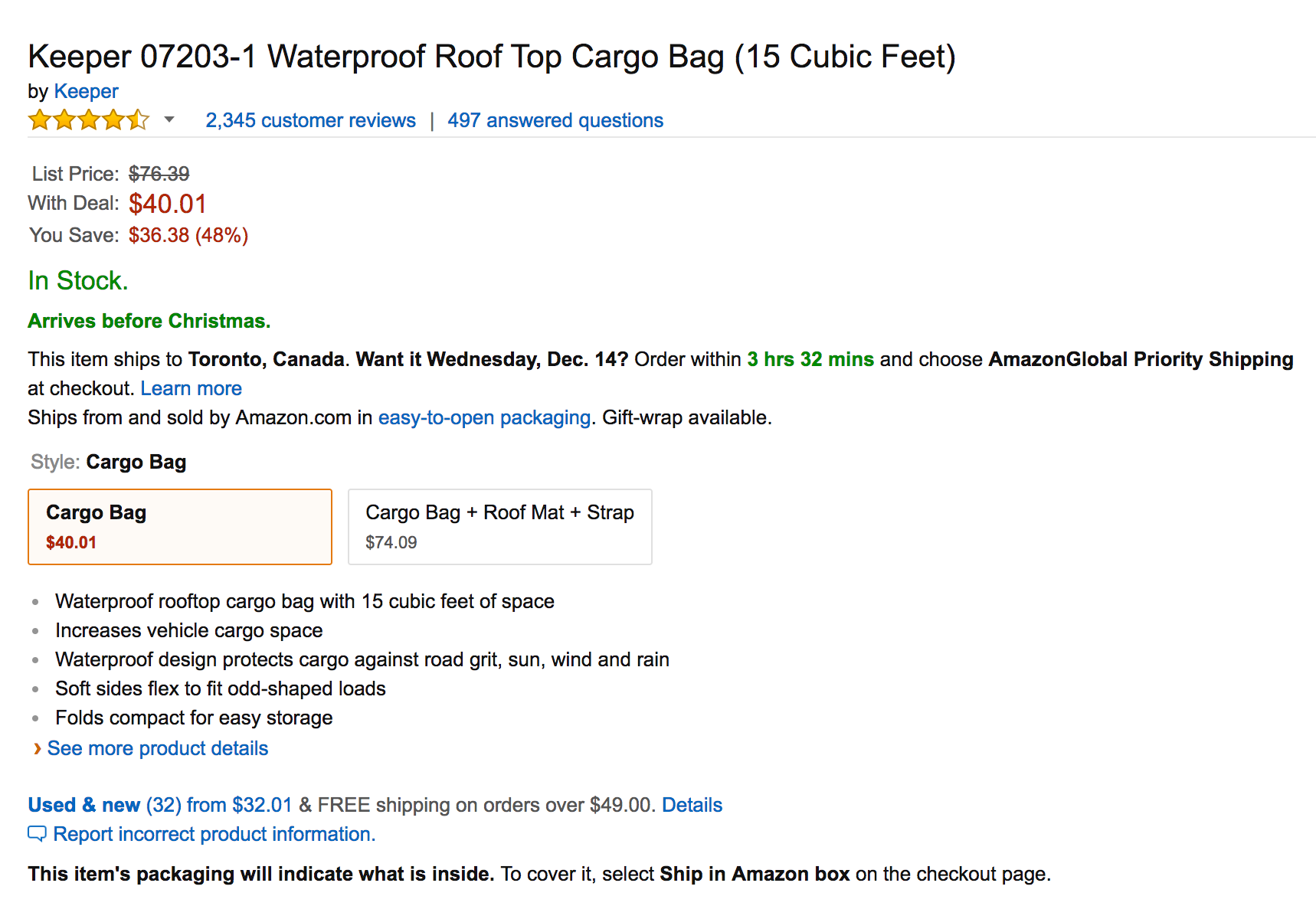This image features a product listing on a white background. At the top, the product is titled "Keeper 07203-1 Waterproof Rooftop Cargo Bag, 15 Cubic Feet" by Keeper. The listing indicates it has an average rating of four and a half stars based on 2,345 customer reviews, and has received 497 answered questions.

The original price of the cargo bag was $76.39, but it is currently available for $40.01, a discount of 48%, saving you $36.38. The listing also notes that the item is in stock and will arrive before Christmas. If shipped to Toronto, Canada, estimated delivery is by Wednesday, December 14th.

The product image shows the cargo bag within a red square. Key features highlighted are:
- 15 cubic feet of storage capacity, increasing vehicle cargo space.
- Waterproof design to protect cargo from road grit, sun, wind, and rain.
- Soft sides that flex to accommodate odd-shaped loads.
- Compact design for easy storage when not in use.

The listing also mentions "See more product details" for additional information. It offers both new and used options, and notes that the item's packaging will reveal its contents. For discreet shipping, customers can select "Ship in Amazon box" at the checkout page.